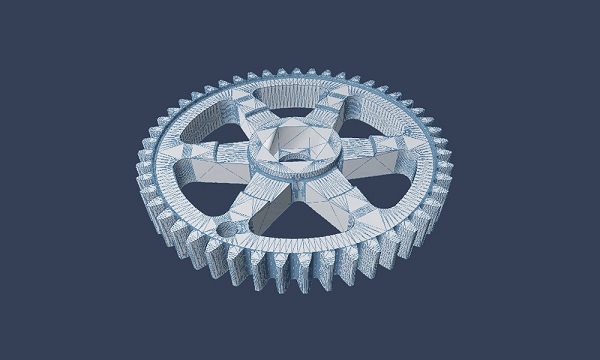The image displays a detailed computer-generated representation of a mechanical cogwheel or gear, set against a very dark blue background. The central area of the gear features a distinctive square shape, which appears to be a hubcap in a silver or gray color. Radiating from this hub are six pointed bars or support beams, extending outward to the cogwheel's spiky, toothed perimeter. The gear itself has a white or light cream base color, intricately etched with blue lines, giving it a textured, 3D appearance. The outer edges of the gear are marked by darker gray, triangular notches, which emphasize its sharp, serrated design. The blue ink detailing adds a striking contrast, making the gear appear to glow lightly against the dark background.